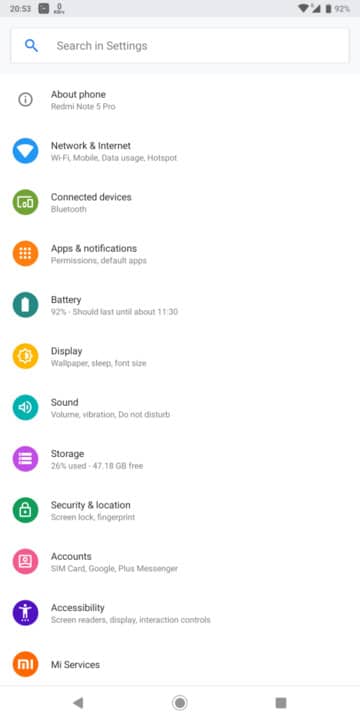In this image, we are presented with the user interface of a phone, likely a Google Play-enabled device. At the top right corner, the screen displays the battery percentage at 92%, accompanied by a battery icon. To the left of the battery icon, we can see the signal strength icon and the Wi-Fi strength icon. On the top left corner, the time is shown as 20:53. 

Just below these icons, there is a rectangular search bar. On the far left of this search bar, there is a blue magnifying glass icon. Positioned slightly to the right, the words "Search settings" are displayed in a light gray color.

Beneath the search bar, there is a vertical list of settings options. The top entry reads "About phone, Redmi Note 5 Pro" with a logo to the left that consists of a circle enclosing an information symbol (i). The next item in the list is "Network & internet," which includes sub-options like Wi-Fi, mobile data usage, and hotspot. Positioned to the left of this setting is a circular icon featuring a Wi-Fi signal strength symbol. 

Continuing down the list, the subsequent entries are as follows:
- "Connected devices" with a Bluetooth icon.
- "Apps & notifications."
- "Battery."
- "Display."
- "Sound."
- "Storage."
- "Security & location."
- "Accounts."
- "Accessibility."

Each entry is neatly categorized with its corresponding graphical icon for easy identification. The clean and organized layout facilitates user navigation through the phone settings.